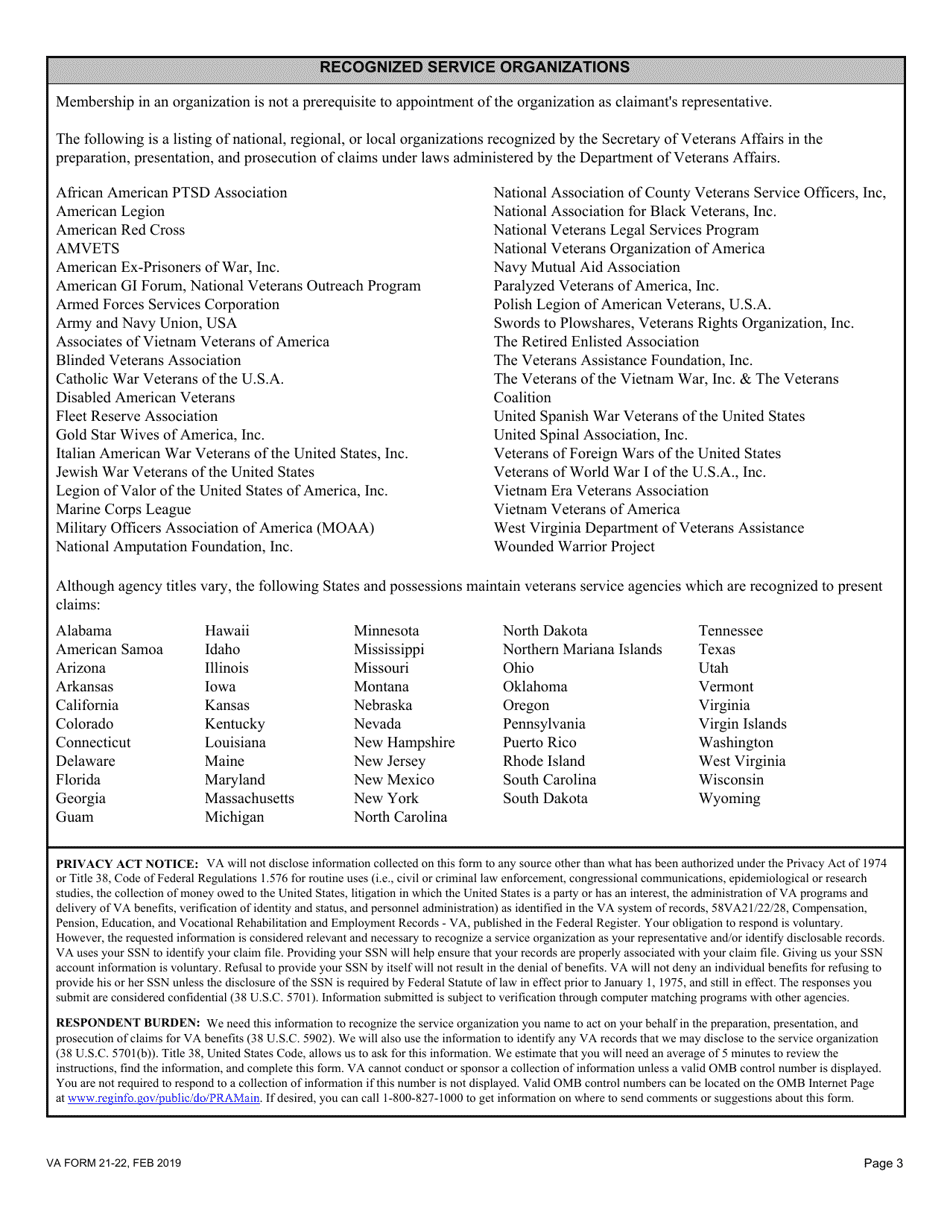This image showcases an official document, specifically Page 3 of the VA Form 21-22 dated February 2019. The document appears to be densely packed with small, closely-spaced text, giving it an official and authoritative appearance likely related to government regulations or procedures. At the top of the page, there is a thin gray bar containing the title "Recognized Service Organizations". Below the title, the background shifts to white with predominantly black text, except for a single blue hyperlink at the bottom.

The central section of the page lists various national, regional, and local organizations recognized by the Secretary of Veterans Affairs for assisting with the preparation, presentation, and prosecution of claims under laws administered by the Department of Veterans Affairs. The text explicitly states that membership in these organizations is not a prerequisite for appointment as a claimant's representative. This list includes a diverse array of organizations, ranging from the African American PTSD Association to the Wounded Warrior Project, totaling over 40 entities presented in two columns.

Further down, the document explains that although organizational titles may vary, all US states and certain territories, including Puerto Rico, maintain Veterans Service Agencies recognized to present claims. The states are listed alphabetically from Alabama to Wyoming.

At the very bottom of the page, in an even smaller font, there is a section titled "Privacy Act Notice" followed by another section discussing "Respondent Burden". A partially legible URL, "www.reginfo.gov/public", is noted in blue text, suggesting an external link for additional information. Overall, the document is intricate and packed with detailed information pertinent to veterans' claim representation.